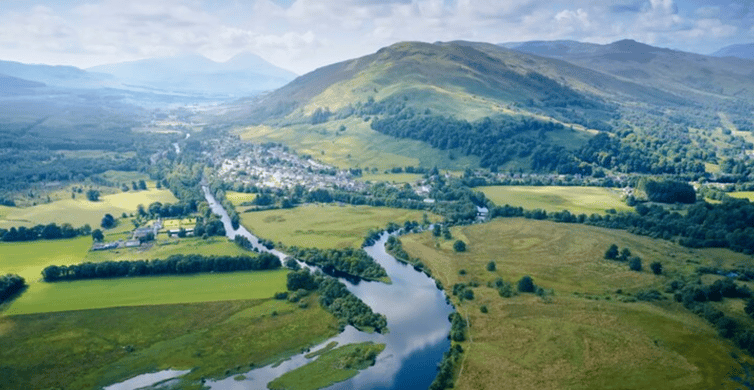This grainy, semi-low aerial photograph captures a serene small town nestled in rolling hills, bathed in the bright, somewhat hazy light of morning. In the bottom left of the frame, a blue river, reflecting the clouds above, curves its way up to the center before branching off to the right. The river also splits sharply to the left, meandering out of the frame and creating a picturesque, meandering water system that flows through the town. Situated at the base of mostly bare hills, the town comprises small, singlestory and two-story white and reddish buildings.

Central to the frame, a solitary copse of trees dots the otherwise bare hillside, while a shallow valley to the right is densely filled with more green trees. The landscape to the left of the river is characterized by bright green rectangular fields, with rows of trees lining the fields. Between two of these fields is a lone building. The land to the right of the river contrasts with short green and brown grass interspersed with sporadic trees.

The wider shot showcases the expanse of the land, including more sloping hills or mountains towards the top right corner, emphasizing the small size and isolation of the village. The general view is rich in greenery, with fields and denser tree clusters providing a verdant contrast to the barren hills.